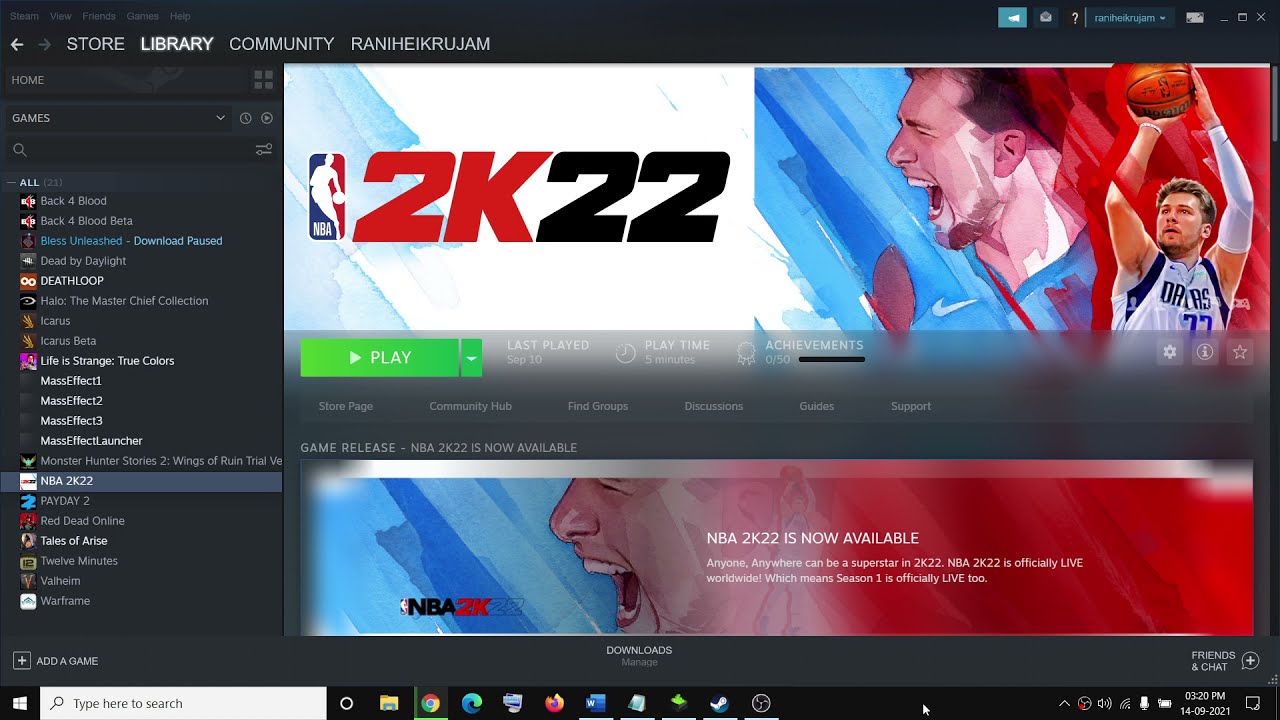A detailed screenshot of a user's Steam interface is displayed. The Steam window features tabs such as Store, Library, and Community, alongside the user's profile name, "raniheikrujam." The profile indicates they own 23 games. Highlighted in the library is "NBA 2K22," showing options to play, with last played date marked as September 10th, and a total playtime of five minutes, with zero achievements unlocked. "NBA 2K22" is noted as newly available, suggesting the screenshot captures its release period.

The user's game collection is presented, listing titles including:
- "Back 4 Blood" and its beta version
- "Dead by Daylight"
- "Halo: The Master Chief Collection"
- "Icarus" and its beta version
- "Life is Strange"
- "Mass Effect Trilogy (1, 2, and 3)"
- "Monster Hunter"
- "Payday 2"
- "Red Dead Online"
- "Tales of Arise"
- "12 Minutes"
- "Warframe"

The operating system is identified as Windows, with the taskbar at the bottom showing icons for Google Chrome, Microsoft Edge, Firefox, Microsoft Word, Notepad, Steam, and two unidentified applications. The date and time displayed are September 14, 2021, at 3:20 p.m. The computer is connected to Wi-Fi, with a fully charged battery.